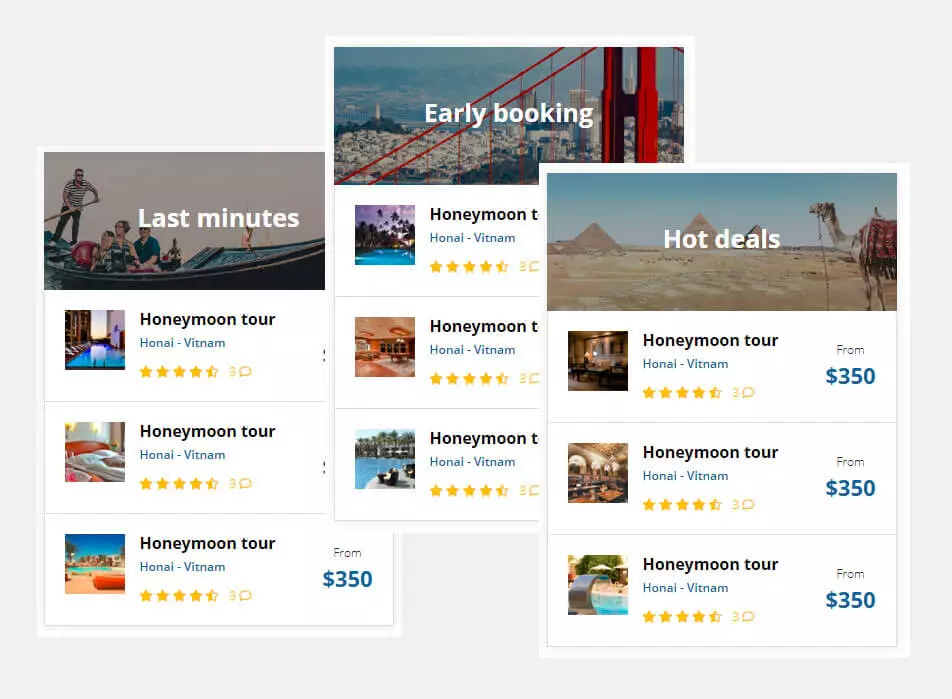The image depicts a webpage from a travel booking site, featuring various deals for hotels and tours. The background is gray, and the page is organized in a grid format, with numerous overlapping boxes showcasing different travel offers. 

In the lower-left corner, a tall white box stands out, topped by a large rectangular picture of a gondola with a chorus in Venice. The gondolier is dressed in a black and white striped shirt, and superimposed white letters read “Last Minute”. Beneath this, three options for different tours are displayed, all labeled "Honeymoon Tour" in black letters. Each option specifies "Hanoi, Vietnam" in blue letters, with a dash separating "Hanoi" and "Vietnam". To the left of these options are three square pictures: the top one appears to show a pool, the middle one a room with white bed sheets, and the bottom one another pool scene beneath a clear blue sky. The price of the bottom option reads “from $350” in blue letters.

The central box is indented at the top, featuring a picture of the Golden Gate Bridge in San Francisco with the city's skyline in the background. White letters in the middle of this picture announce "Early Booking". Below, the same "Honeymoon Tour" labels and "Hanoi, Vietnam" details are repeated, each accompanied by five stars (the fifth star partially filled in) and a yellow number "3" with a speech bubble icon next to it. The box also displays three squares: the top one shows a sunset scene with palm trees by a pool, the middle one depicts the interior of a hotel lobby with wooden floors, and the bottom one captures another poolside view, though the details are small and indistinct.

To the far right, a long rectangular image showcases the pyramids in Egypt, with "Hot Deals" text in the middle. A camel is visible to the right of the pyramids. Below this, identical "Honeymoon Tour" and "Hanoi, Vietnam" labels are shown, along with the same star ratings and speech bubble icon. Prices labeled “from $350” in blue letters are repeated here as well. The accompanying square images, though small and difficult to discern, seem to depict interior scenes, likely from restaurants or dining areas, with one picture possibly showing a pool scene with a silver diving board.

Overall, the webpage appears to be a landing page for a travel booking site, showcasing various deals and options in a visually intricate and overlapping format.